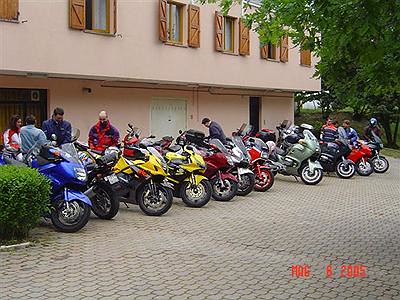The photograph captures an outdoor scene of a cobblestone parking lot in front of a two-story pink stucco building with wooden shutters on the windows. Lined up in a row, facing the same direction, are eleven sport bikes in a variety of colors including blue, yellow, red, green, black, silver, and possibly orange. These bikes all have their front wheels and parts facing forward, indicating a meetup or gathering. People, mostly men, are milling about, with one woman visible and one person wearing a helmet, suggesting they might own one of the bikes. The time stamp at the bottom of the picture is blurry but indicates a date in August 2005. The scene includes additional details like an open area of brush and a cement block, set against what appears to be a cloudy day.